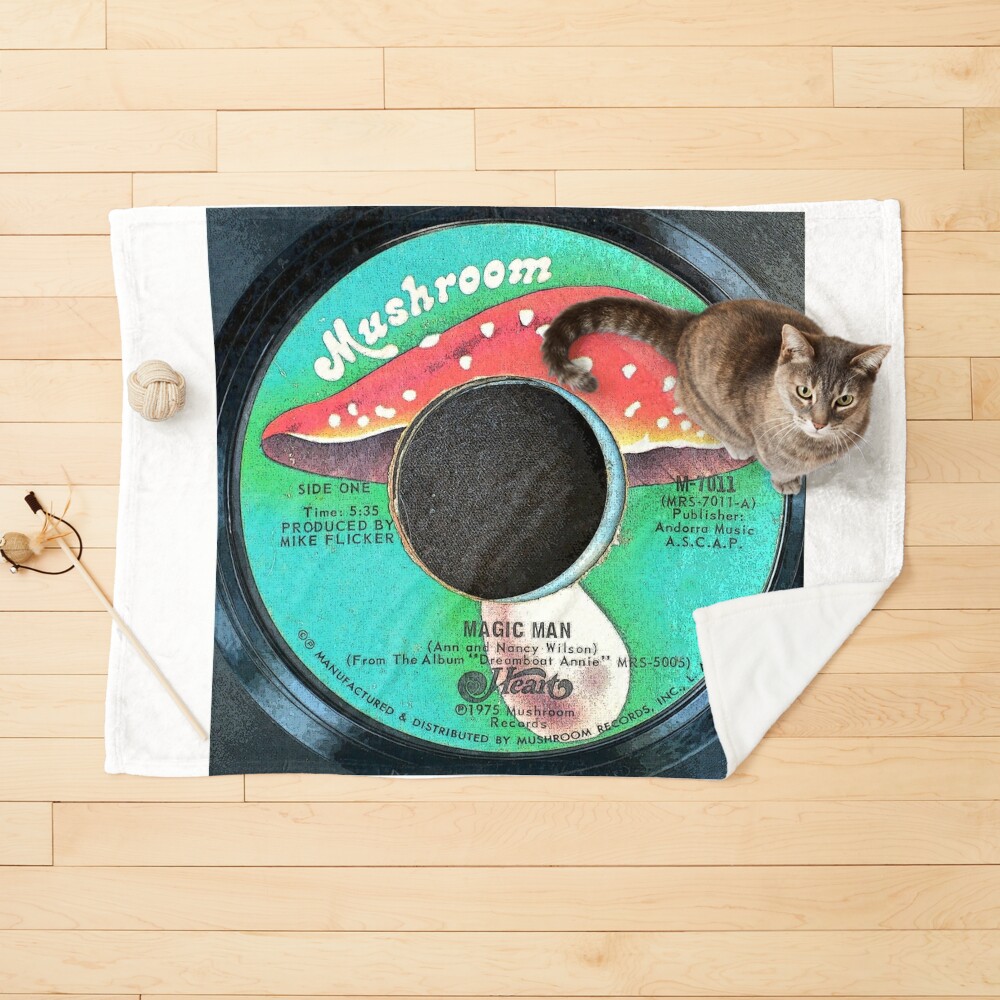This photograph, taken from a vertical angle, captures a light beige wooden floor with a rug designed to look like an old 45 record cover. The rug features a black center with the word 'Mushroom' written in a white, 60s-style font and a drawing of a red-capped mushroom. The title 'Magic Man' is displayed prominently, along with 'Side 1, produced by Mike Flicker,' and mentions Anne and Nancy Wilson from the album "Dream Boat Annie" (1975) by Heart. The corner of the rug on the bottom right is flipped up. A gray cat is standing on the upper right side of the rug, looking up at the camera. To the left of the rug, there are a couple of cat toys: a small ball of yarn and a wooden wand with feathers and dangling items. The photograph captures a moment of the cat's curiosity, juxtaposed with the nostalgic design of the rug that mimics the iconic record.